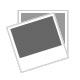This photograph showcases a detailed framed painting of a dramatic ocean scene featuring rocky cliffs and crashing waves. The green water flows through a narrow passage between two prominent brown and yellow rocks, which have patches of grass or plants on top. In the center of the water, a rock outcropping faces the impact of the waves, causing them to splash upward. Above, a light blue sky with sparse clouds adds to the scene's tranquility. The painting is encased in an exceptionally ornate and elaborate gold frame, consisting of multiple intricate borders that include layers of brown, black, and golden interlocking designs.